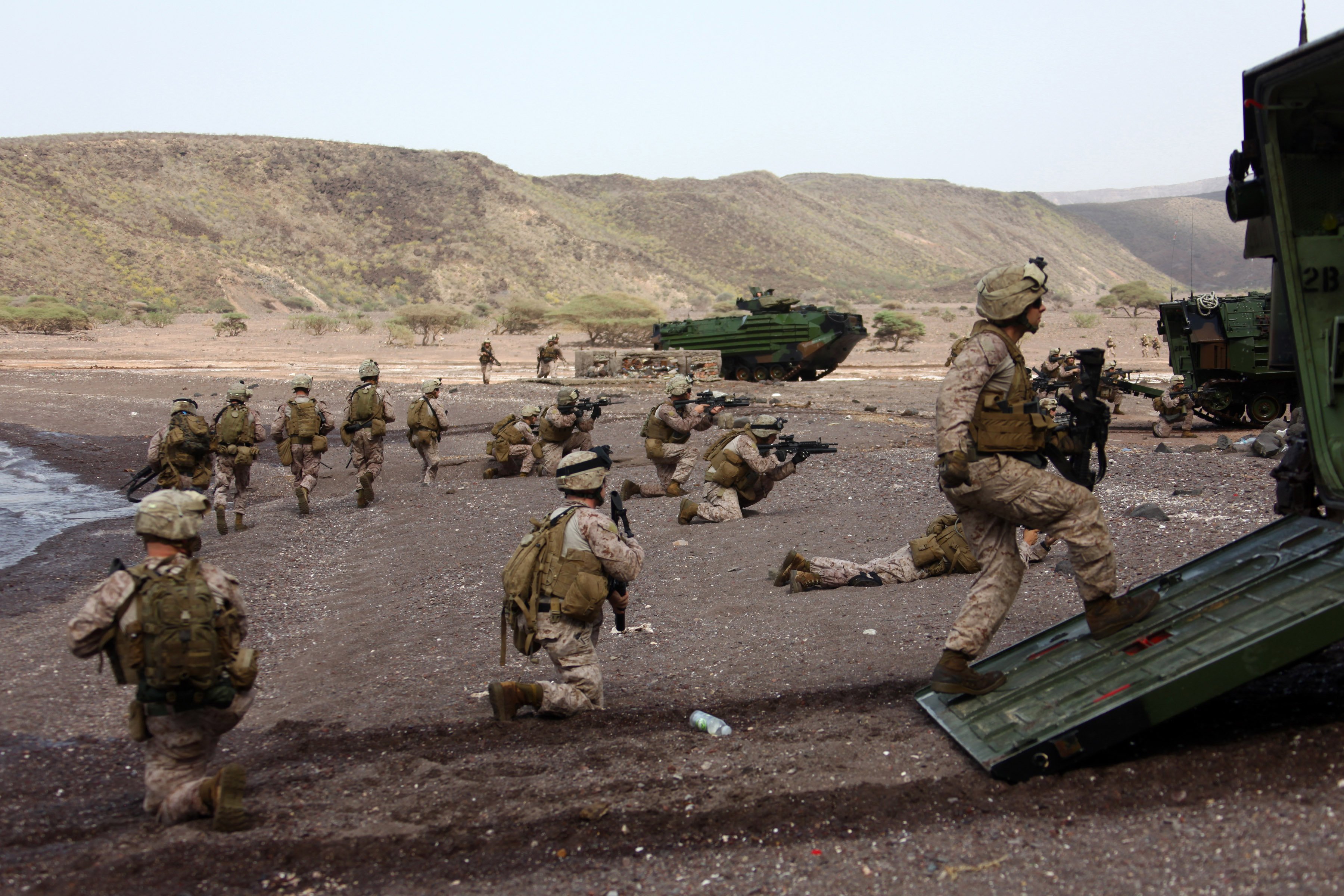In this horizontal photograph, a dozen soldiers are engaged in what appears to be a military training exercise or possibly a real operation in an outdoor, dirt-covered area near a shoreline. The scene is set against a backdrop of green hills and distant mountains. The soldiers, dressed in desert camo uniforms with darker brown vests, are primarily kneeling on the ground, aiming their black rifles. Some soldiers are standing, while a few are walking or jogging towards an open, green armored vehicle with its back door ajar. A green helicopter is positioned near the soldiers, and additional military trucks or vehicles can be seen in the far background. The overall tone of the image suggests a coordinated military maneuver in a rugged, natural landscape.